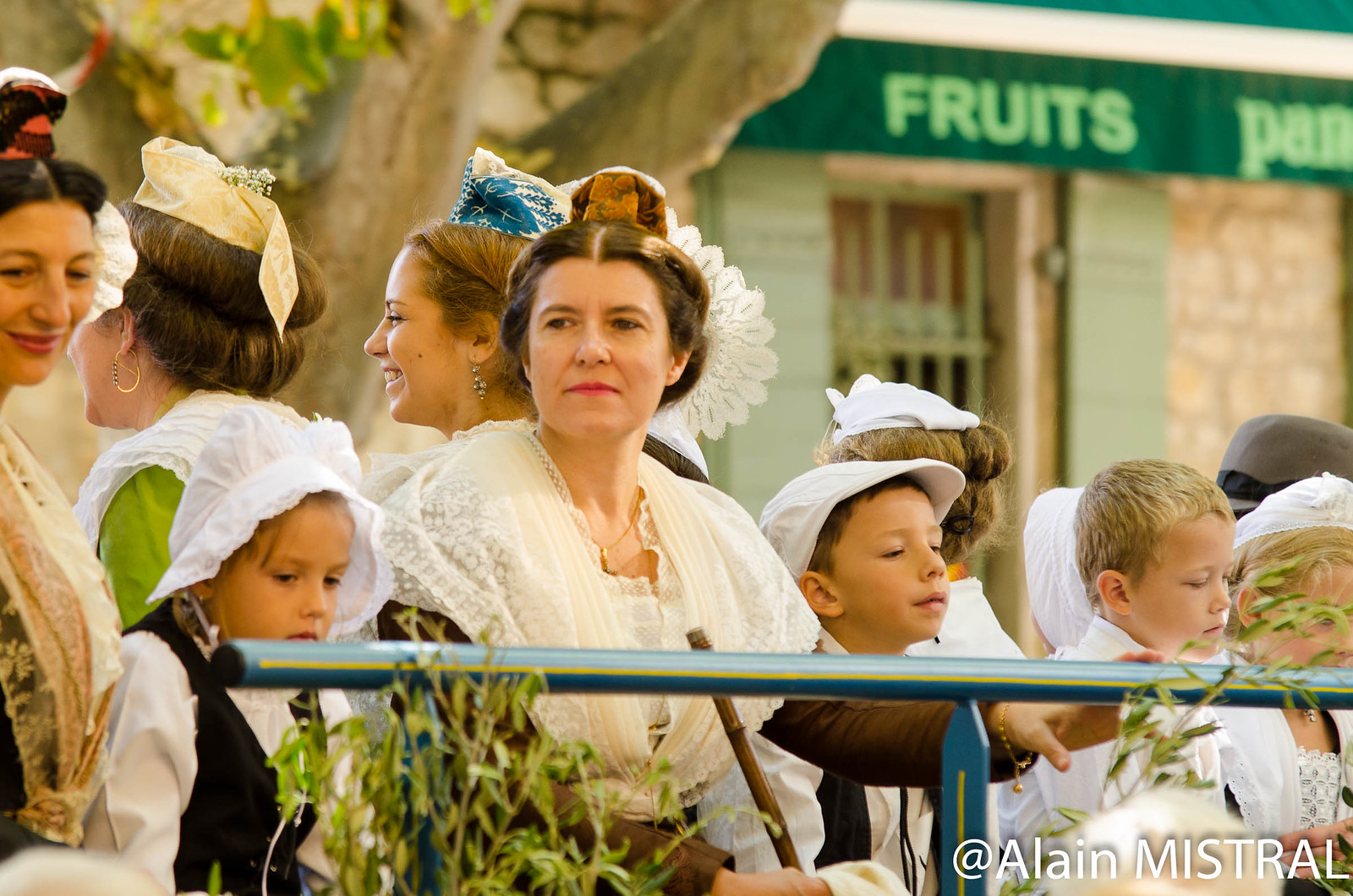A detailed photograph captures a group of Caucasian women and children clad in period costumes reminiscent of the early 1800s. The children, nearly all wearing white caps or bonnets, are accompanied by a few boys, one of whom is hatless. The women are elegantly dressed in lacy shawls with their hair styled in buns and capped with delicate headpieces, one of which is notably bluish. They stand behind a blue metal railing, suggesting a parade route or a similar public gathering. Prominently in the background, a green banner on the storefront behind them reads "Fruits," situated next to a brown door. Additionally, a green shrub is visible in the foreground. The bottom of the picture contains an inscription, "Allian Mistral," linked to the photograph's context.